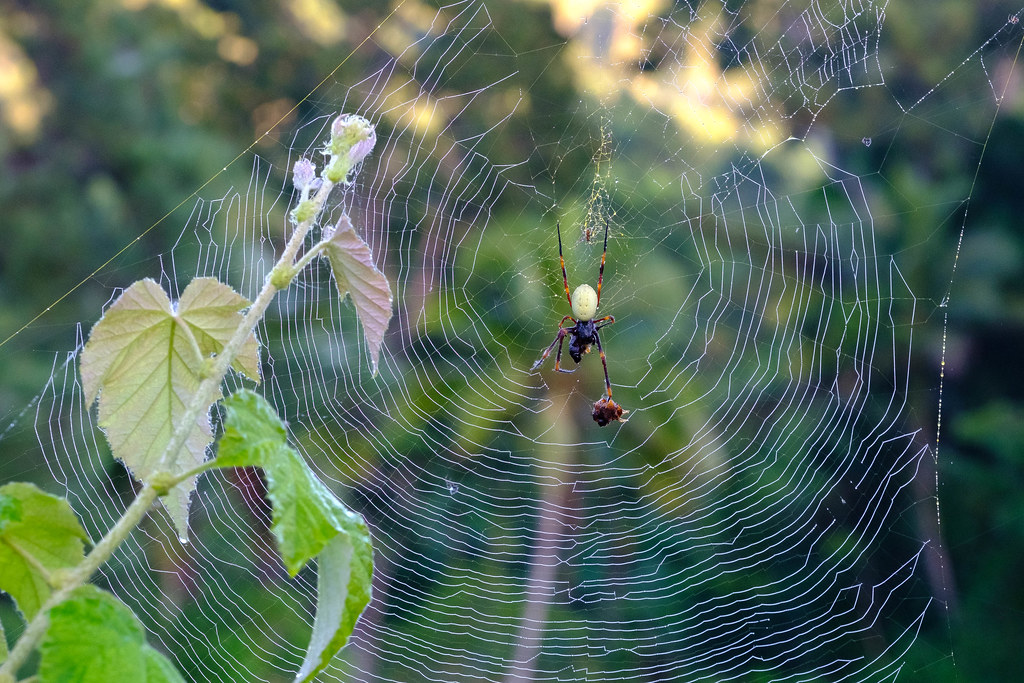This is a detailed close-up photo of an orb weaver spider navigating its expansive white web during the day. The spider, with a distinctive yellow abdomen and brown legs featuring black tips and sections, is prominent in the center of the image. One of its right legs is making contact with an insect that has been ensnared in its web, indicating a recent capture. There is intricate detail in the spider's coloration, which includes hues of orange and possibly navy blue. The web is strategically attached to a plant with light green leaves, one of which shows a forest green underside. The plant's stem extends upwards, slightly flowering with delicate pink blooms at the top. The background is an unfocused blend of forest foliage, predominantly green, with sunlight piercing through. Additionally, a blurred tree branch can be seen on the left side of the composition. The vibrant colors present include green, white, purple, yellow, gray, and orange, creating a rich and dynamic visual.